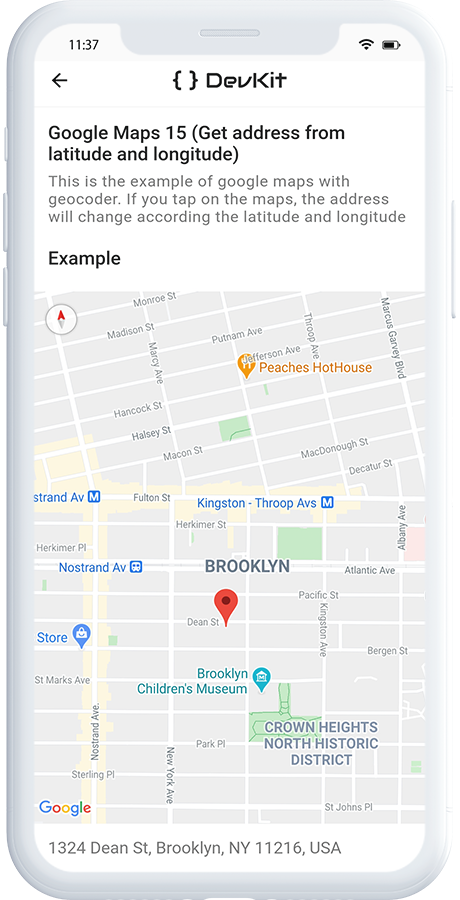In this image, we are looking at a screenshot from a white cell phone, showcasing a Google Maps interface. The phone features two equally-sized buttons on the left side with a smaller button above them, and a single button on the top right side. The background is white.

The status bar at the top-left corner displays the time as 11:37 and shows that Wi-Fi is connected and the battery is nearly full. Below this, in bold black text, is the line "Google Maps 15. Get address from latitude and longitude."

The interface demonstrates an example of Google Maps with Geocoder functionality. If you tap on the map, the address will change according to the specified latitude and longitude. Below this description, also in bold black text, is a visual example on the left, showing a map that is primarily gray. A red pin marks a location labeled "Dean Street" in Brooklyn. This location is situated just above the Crown Heights North Historic District and the Brooklyn Children's Museum, and below Kingston-Throop Avenue.

At the bottom of the screen, there is a white search bar showing the address "1324 Dean Street, Brooklyn, New York".